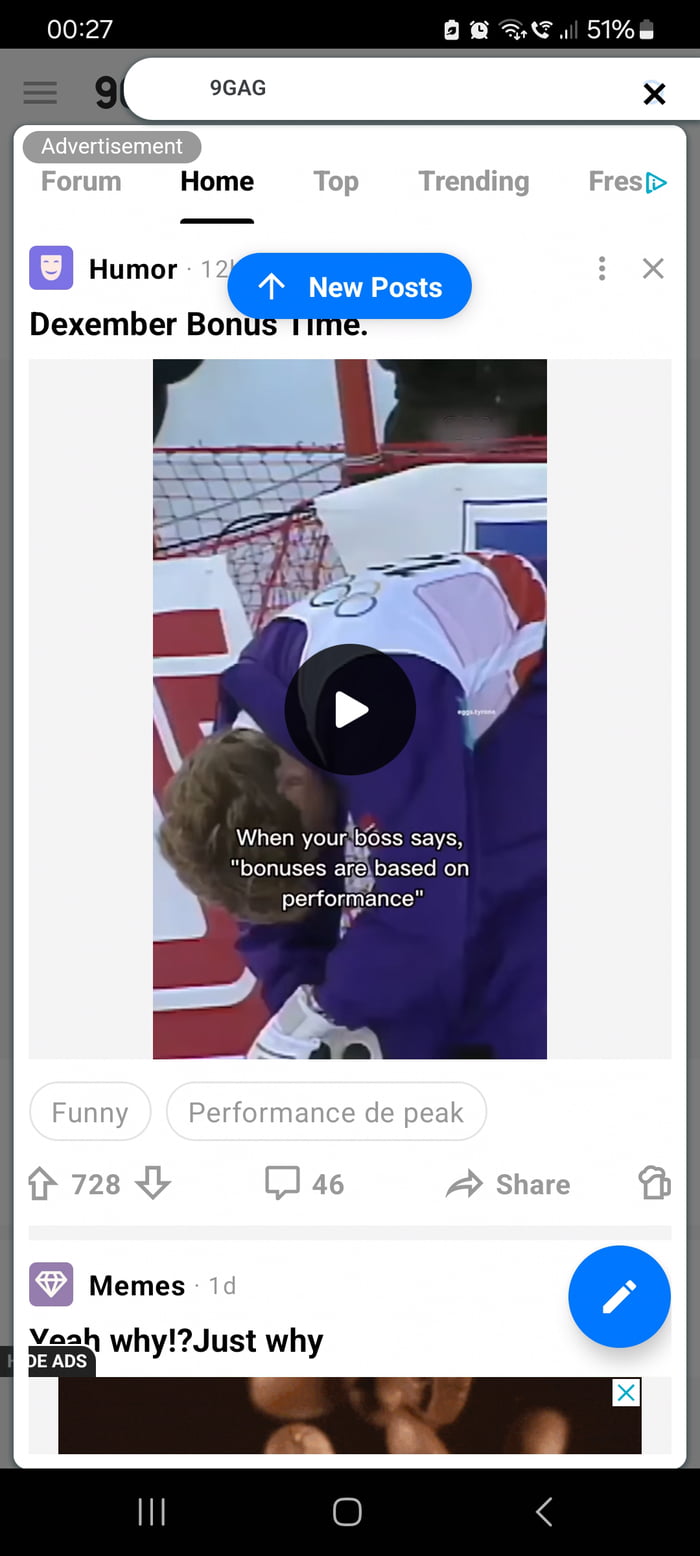The image is a screenshot taken from the 9GAG app, captured at exactly 00:27, as indicated on the top black bar. This bar also displays various icons on the right side, such as battery health, an alarm clock, signal strength, and battery percentage.

Central to the screenshot is a search bar, positioned slightly to the right, which reads "9GAG" with an 'X' for closing it. Directly below the search bar is a notable white rectangle with a centered image of an Olympic athlete. The athlete, who has short brown hair, is wearing a jacket featuring the Olympic symbol on the back and is bent over at the waist with their hands reaching down. A net is visible in the background, providing context for the setting.

This post falls under the 'Humor' section on 9GAG and there is an arrow for navigating to new posts, marked with "December bonus time." Embedded within the Olympic athlete image is a play button, signifying it’s a video. Overlay text on the screenshot reads, "When your boss says bonuses are based on performance."

Below the main content, the post shows engagement metrics: 728 upvotes, an unspecified number of downvotes, and 46 comments. There are options to share the post and a small beer icon likely representing a fun or celebratory action.

Partially visible below this post is another image mainly black with tan circles, likely suggesting a hand. The title of this next post in the meme section is "Yeah why, just why." At the bottom of the screenshot are options including an edit button, along with icons for the phone’s menu, app searcher, and back button.